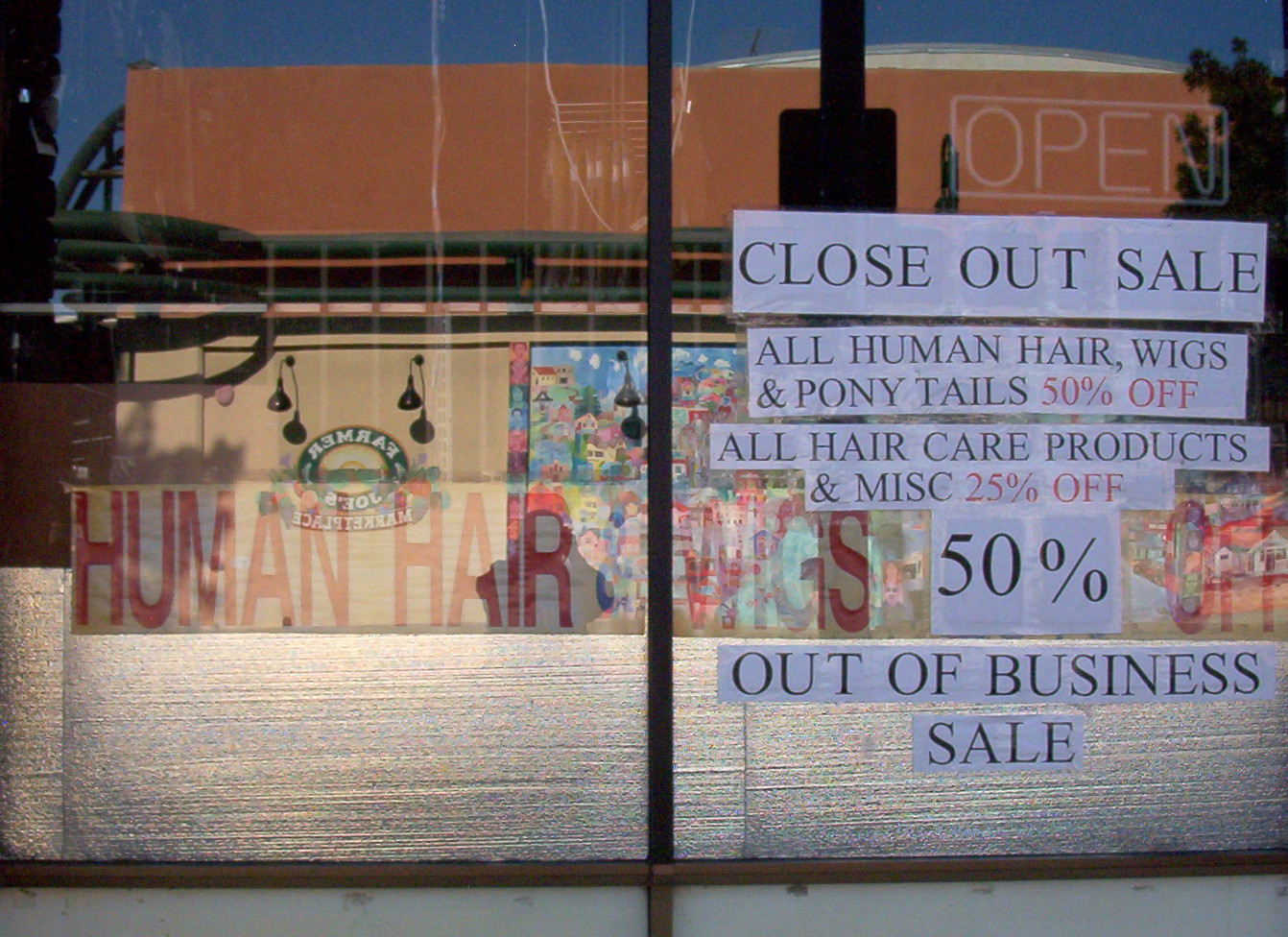This photograph showcases the front of a store with large glass windows. Reflected in the glass is a red brick building and the "Farmer Joe's Marketplace" logo from across the street. The storefront is divided in half by a metal framework. The left window features a prominent white banner with red capital letters stating "Human Hair." Spread across both windows, various signs detail the store's sales: a closeout sale offering all human hair, wigs, and ponytails at 50% off, and all hair care products at 25% off. A large sign below highlights a "50% Out of Business Sale." In the right window, an unlit "Open" sign is visible. The clear reflections also show additional building details and lamps from the surroundings.